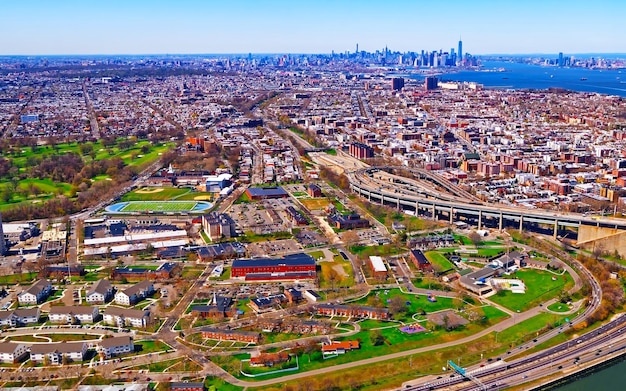This color aerial photograph captures a vibrant urban landscape, most likely New York City, with New Jersey in the immediate foreground. The foreground features a compact, suburban sprawl characterized by housing developments, a school, and areas of greenery interspersed with trees. To the middle left, a section of grass and trees adds a touch of nature amid the urban chaos. Prominent road infrastructure, including a complex highway system, a bypass, and an interstate, weaves through the scene, connecting various residential and business areas. A football field and a baseball field are also visible.

In the midground, the density intensifies with a mix of mid-rise buildings filling up the space between the more suburban area and the distant cityscape. The skyline of Manhattan dominates the background, with the One World Trade Center standing out prominently among the other towering skyscrapers. Stretching to the right of the cityscape, water adds contrast to the urban density. Every inch of the photograph is filled with either buildings or infrastructure, underscoring the city's bustling, congested nature. Despite the graininess, this photograph vividly illustrates the complexity and scale of the metropolitan area.